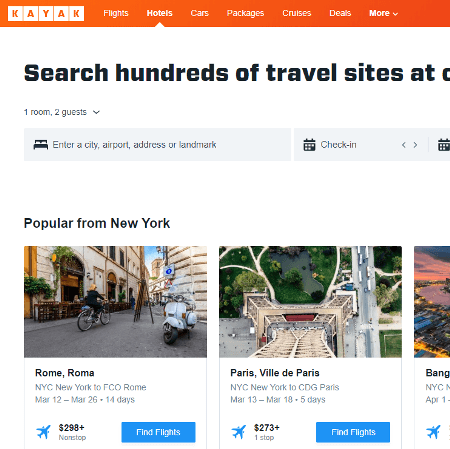The image shows a screenshot from the Kayak travel booking website. At the top, there's a navigation bar offering various booking options such as flights, hotels, cars, packages, cruises, and deals. Below the navigation bar, a search area allows users to input their travel destination, check-in and check-out dates, and the number of guests.

The main section of the page prominently features popular travel destinations departing from New York. Each destination block, showcasing a beautiful image and a brief description, includes options to find flights. Notable destinations visible in the image are Rome, Italy (with available travel dates from March 12th to March 26th), Paris, France (from March 13th to March 18th), and Bangkok, Thailand (on April 14th). The dates for Bangkok destinations are partially cut off in the image.

Overall, the screenshot captures Kayak's user-friendly design, enabling users to easily discover and book travel options to their desired locations.